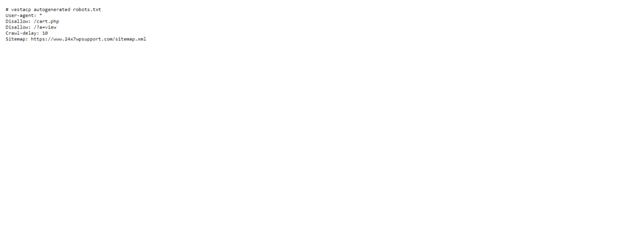In this image, the focus is on an extremely small block of black text located in the top left corner against a white background. The text consists of six lines. The top line contains four words, followed by a second line with two words. The third line has three words, the fourth line two words, and the fifth line three words. The final line features a single word accompanied by a website link. The text is so small that it is difficult to discern the exact content. The rest of the image is a plain white background, emphasizing the tiny, unreadable text in the corner.